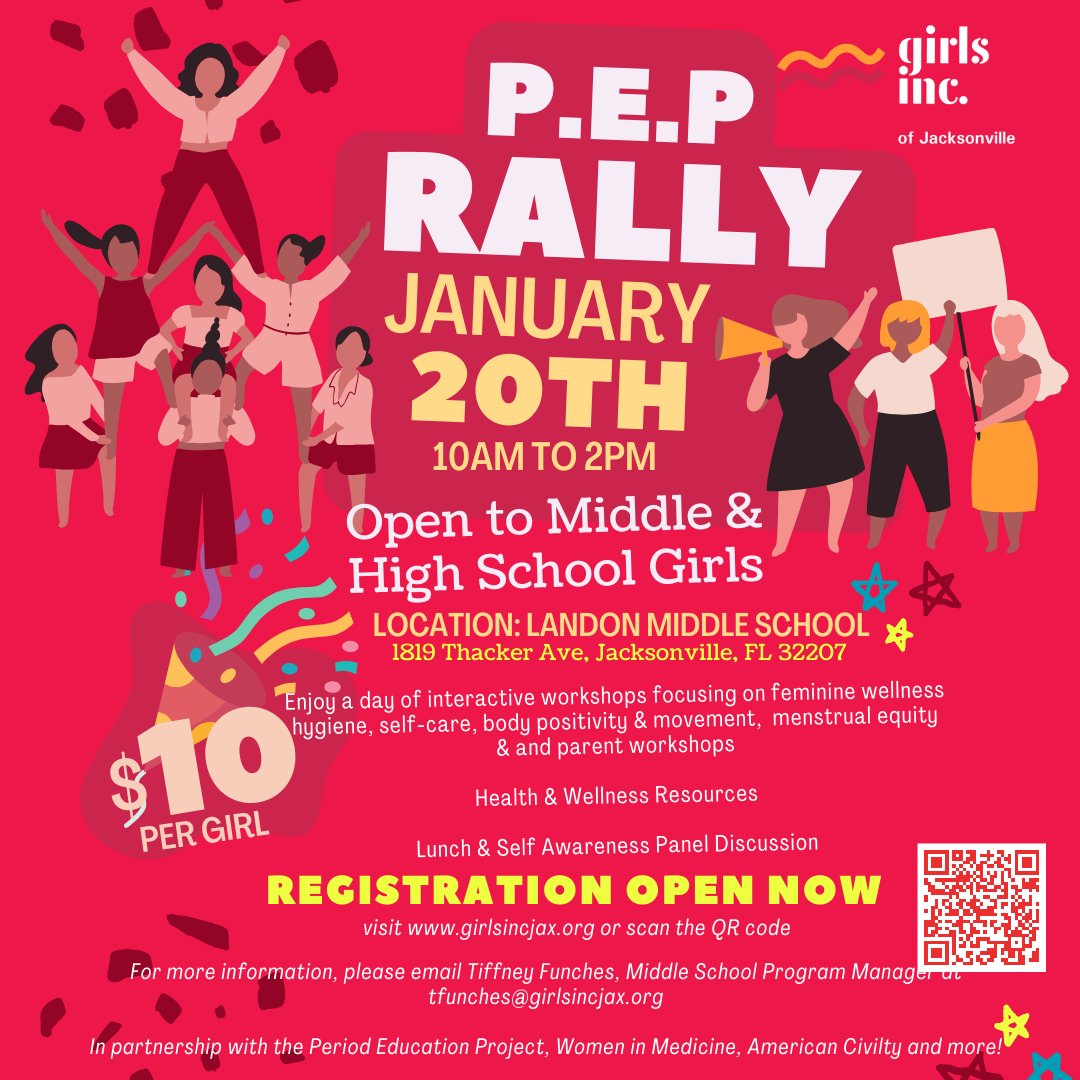The poster for the upcoming event, organized by Girls Inc. of Jacksonville, prominently displays a vibrant red background featuring six cartoon-style women without detailed faces. These figures are dressed in various combinations of red and pink attire. At the top right, the text "Girls Inc. of Jacksonville" is clearly visible. The event, titled "Pep Rally," is scheduled for January 20th from 10 a.m. to 2 p.m. at Landon Middle School, located at 1819 Thacker Avenue, Jacksonville, Florida, 32207. 

Middle and high school girls are invited to participate for a fee of $10 per person, which includes a party favor. The day will be filled with interactive workshops that focus on feminine wellness, hygiene, self-care, body positivity, and movement. Additionally, there will be sessions on menstrual equity and parent workshops, along with health and wellness resources. Attendees can enjoy lunch and a self-awareness panel discussion. 

The poster highlights that registration is now open, with instructions to visit www.girlsincjacks.org or scan the adjacent QR code. For more information, Tiffany Funches, the Middle School Program Manager, can be contacted at tfunches@girlsincjacks.org. This event is presented in partnership with the Period Education Project, Women in Medicine, American Civility, and other organizations.